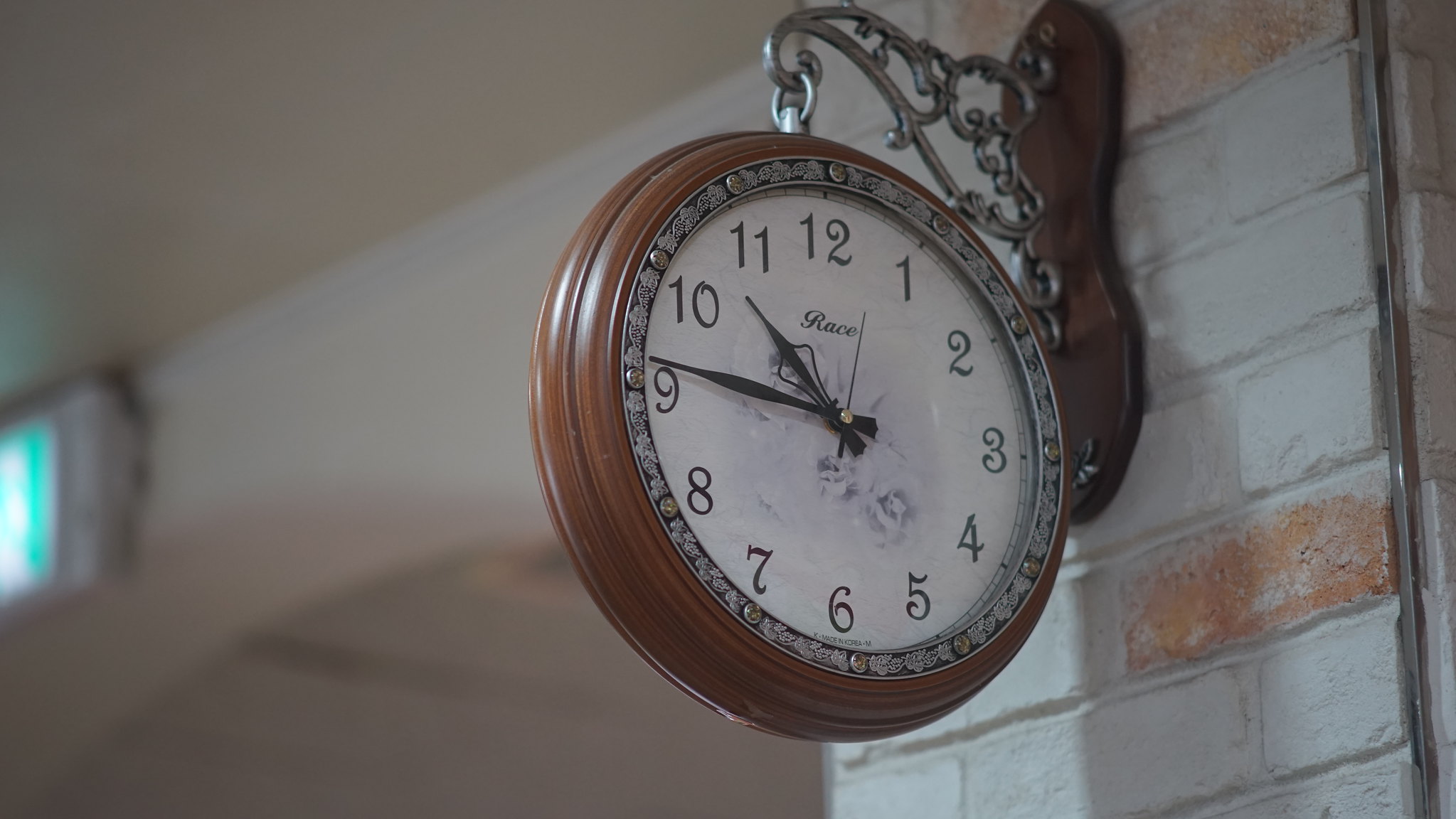This image depicts a clock mounted on the exterior of a building. The clock is affixed to a brick wall that is painted in a light gray color. The paint on the wall is weathered, revealing patches of the original red brick underneath. The clock is secured to the wall via a wooden plaque, which is attached to the brick surface with staples or nails. Extending from this plaque is an intricate metal bracket that supports the hanging clock.

The clock itself appears to be crafted from wood, exhibiting a brown frame. Encircling the white clock face is a decorative layer of stones. The clock face features bold black numerals from 1 to 12 and black hands indicating the time as 10:47. The center of the clock face has the word "RACE" prominently displayed. Judging by the brightness in the surrounding environment, it is likely that the image was captured during daytime, suggesting it is 10:47 AM.